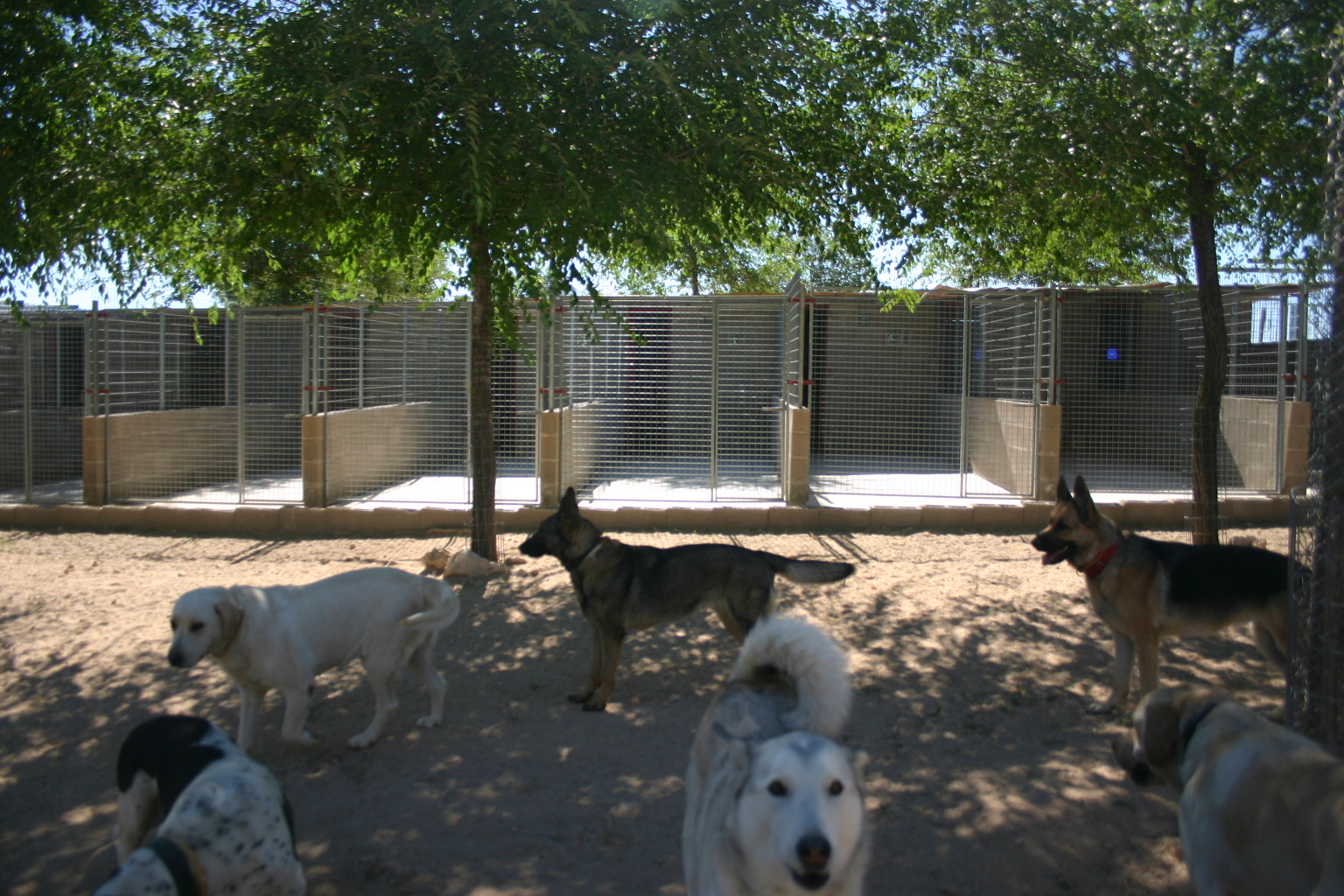The photograph captures a daytime scene at an outdoor dog boarding facility, showcasing a structured and well-maintained environment for the dogs. In the background, there are several large dog kennels, each with wire doors on the right side. The kennels are divided by stone ledges at the base, with wire fences forming the top half and fully enclosing them like mini rooms or stalls. The area is shaded and well-lit, as evidenced by the trees evenly spaced in front of the kennels, displaying lush green leaves. 

In the foreground, there are six large dogs of various breeds standing around on a dirt or sandy ground. The group includes two German Shepherds, a Golden Retriever, an Australian Shepherd, a silver and white dog, and a brown dog with drooping ears. The scene reflects a calm and organized setting, ideal for the dogs to move around and interact within their shaded outdoor shelter.